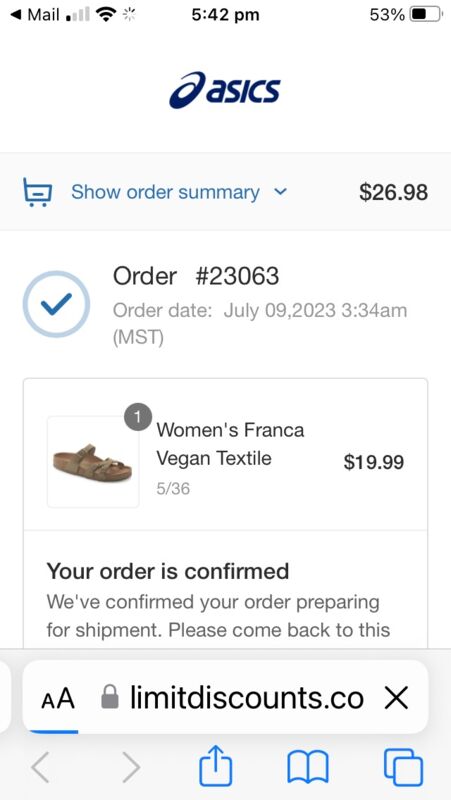Screenshot of a smartphone display showing a confirmation page for an online order. The device is connected to Wi-Fi with one bar, and the current time is 5:42 p.m. The battery is at 53%. The webpage belongs to Hasek's, with their logo prominently displayed. 

On a gray background, blue text reads "Show order summary" with a small cart icon to the left and a down arrow. The order total of $26.98 is displayed in black text. Below, a light blue circle with a blue checkmark denotes successful order placement. 

The order details show a white background with black text: 
- Order number 23063
- Order date: July 9th, 2023, 3:34 a.m. MST

A gray-outlined box contains an image of sandals with a small gray circle indicating the quantity of one. The product description reads "Women's Franca Vegan Textile, size 36, $19.95". Below the image, a notification states: "Your order is confirmed. We've confirmed your order and are preparing it for shipment. Please check back for updates."

At the bottom of the screen, there is a link to limitdiscounts.com.